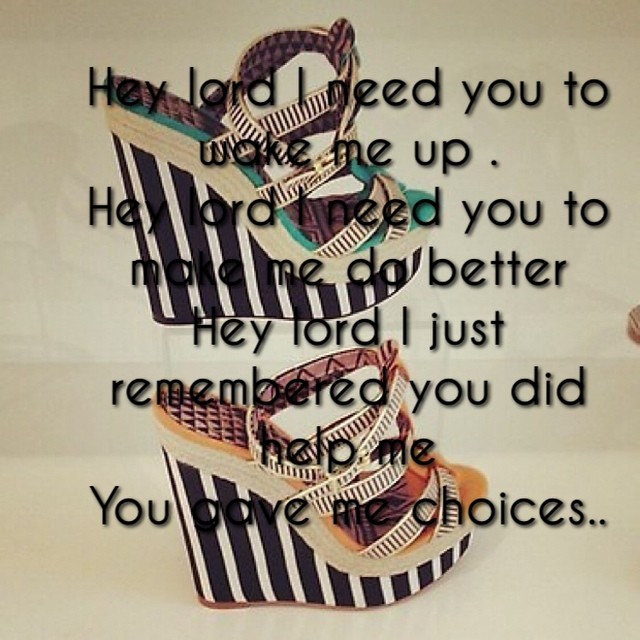The image is a flyer featuring a drawing of two high-heeled platform sandals stacked on top of each other against a yellowish-brown paper background. The heels of the shoes are adorned with black and white stripes. The sandal at the top has brown and green accents, while the bottom sandal has reddish-brown and light orange accents. A black text overlay, resembling an embossed texture, runs across the image, making it somewhat difficult to read due to the colorful background. The text reads, "Hey, Lord, I need you to wake me up. Hey, Lord, I need you to make me do better. Hey, Lord, I just remembered you did help me. You gave me choices..." There are no other graphic elements in the image, giving it an inspirational and motivational tone typical of meme-style posts.